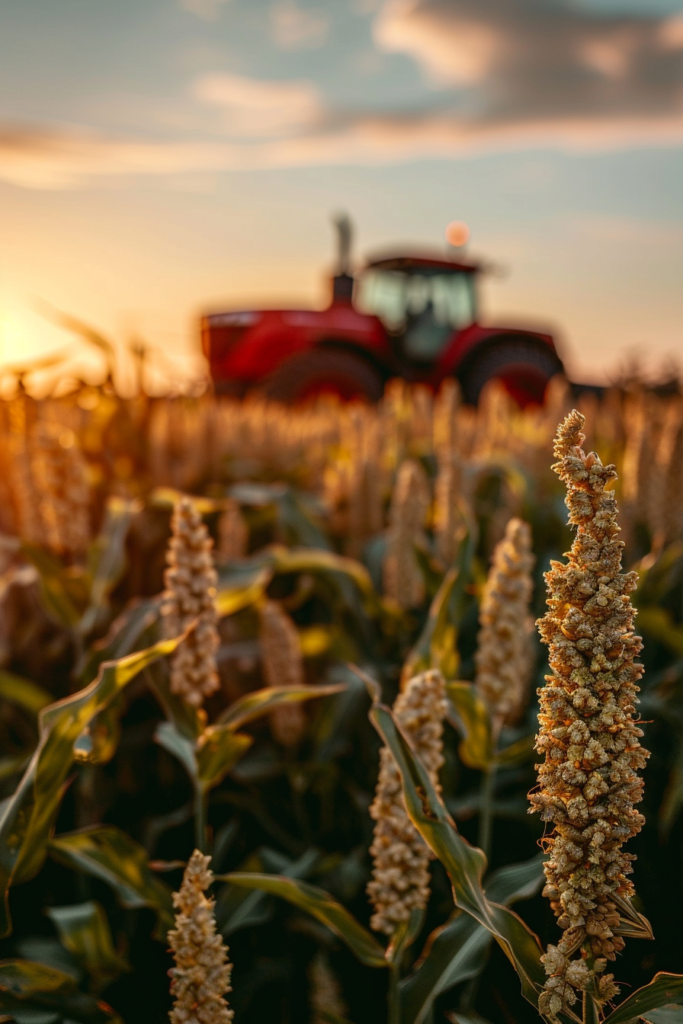The image is a detailed, close-up color photograph of a wheat field taken during daylight. In the foreground, the tops of the wheat stalks are in sharp focus, revealing their long, thin brown and yellow heads composed of many small independent grains. The tall green stems with broad leaves are identifiable beneath the grain heads. The field stretches out into the background where the stalks become increasingly blurred, blending into a tapestry of yellowish hues.

Towards the left of the mid-ground, there is a large red tractor partially obscured by the depth of field effect, featuring a yellow light at the top and a smoke stack. The tractor appears to have an enclosed cabin and is facing to the left. The scene extends into the distant background where the entire field fades into a blur, capturing the expanse of the agricultural landscape.

Above this field, the sky is a light blue with dark overcast clouds, suggesting either early morning or late evening light. The sun is subtly indicated on the far left horizon, potentially rising or setting behind the clouds. The overall composition blends both sharp and softened elements to give a sense of the vastness and serene atmosphere of the rural setting.